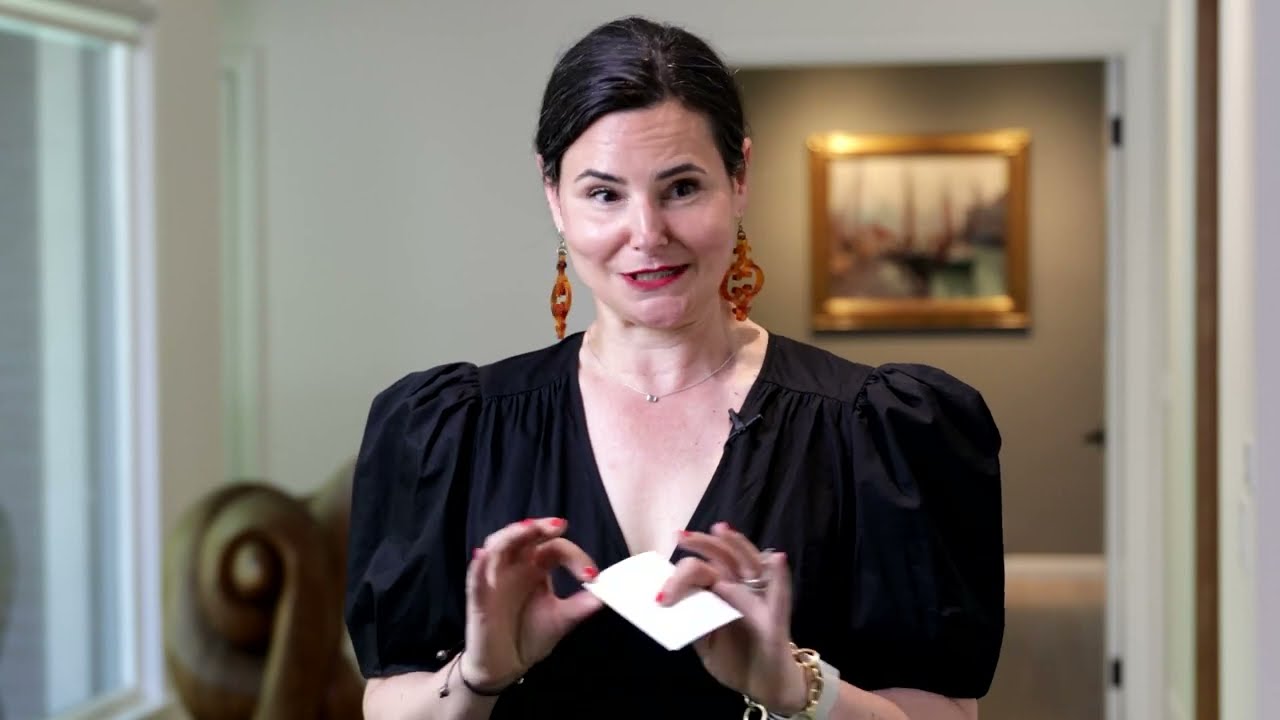This image captures a middle-aged woman, likely in her 50s, who is centered and holding a note or card while looking down to the right, giving the impression that she is listening to someone. She has dark hair pulled back, displaying her large, dangly earrings in shades of red, purple, and gold. She is wearing a black dress with puffy sleeves and a low-cut neckline, complemented by red nail polish and a gold necklace featuring a white pearl. Both of her wrists are adorned with multiple bracelets, including a white watch on one arm.

In the background, there is a slightly out-of-focus beige wall with a gold-framed picture that appears to depict ships. On the right side of the image, there are door hinges and a white wall with brown trim, suggesting an open door. To her left, there is a window, and a brown couch is visible directly behind her, creating a cozy, possibly domestic setting. This scene, which could resemble a moment from a reality TV show, conveys a mix of elegance and everyday life.